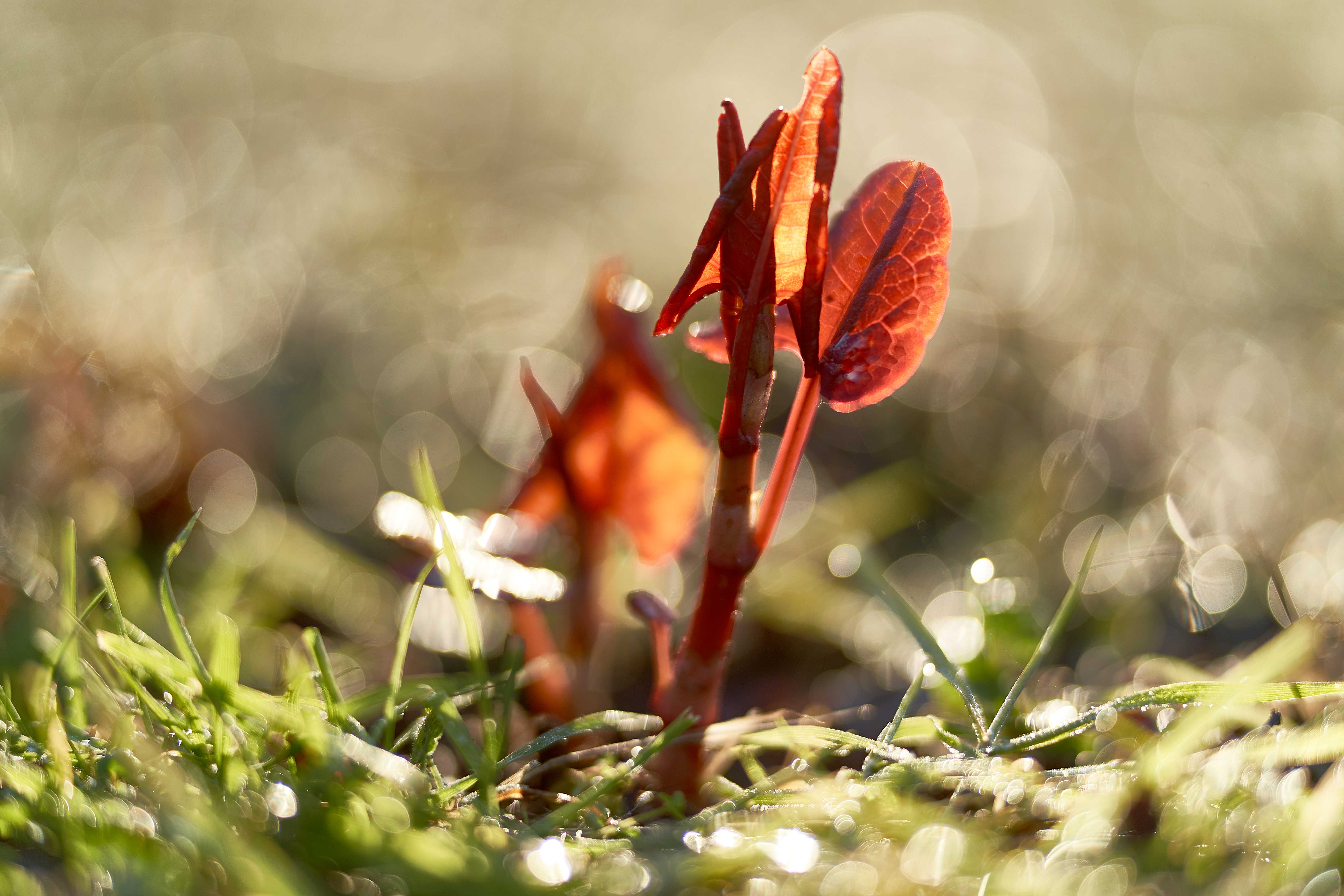The image is a close-up of a young red plant sprouting from a grassy field. The plant features a thick red stalk with slightly lighter stripes along its sides. From the bottom of the stalk, a branch extends, ending in a blue bulb. The top of the plant displays two arrow-shaped leaves, while a rounder leaf emerges from its right side. The surrounding grass appears wet, possibly from morning dew, and hints of sunlight reflect off the ground. The overall scene, captured on a sunny day, highlights the plant emerging through dark green, wiry grass, accompanied by a few scattered clovers. The sunlight illuminates the red leaves, giving them a translucent appearance.